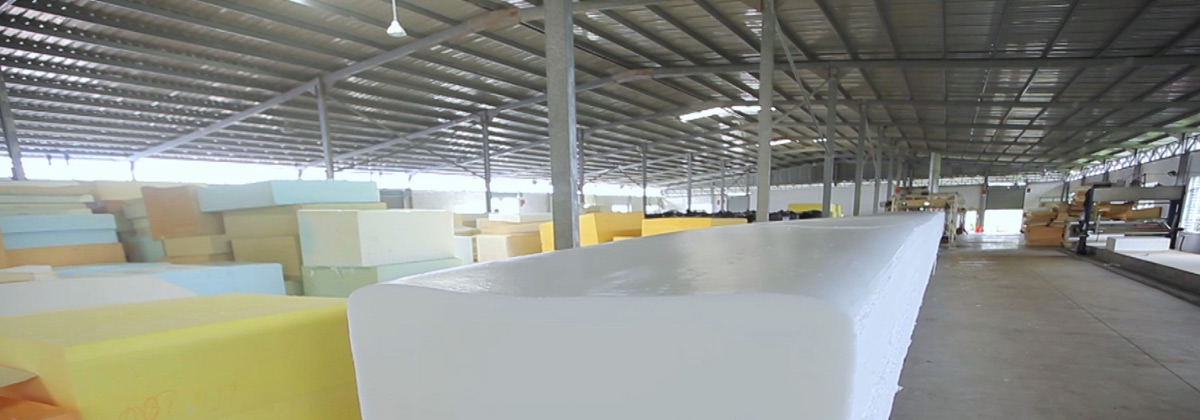The image depicts the interior of a spacious warehouse with a metallic roof supported by numerous steel girders and posts. The floor is made of concrete, adding to the industrial feel of the setting. Scattered throughout the warehouse are large rectangular and cube-shaped objects that appear to be made of foam or styrofoam, judging by their bulky and somewhat amorphous appearance. These objects come in various colors, including gray, brown, white, yellow, light blue, green, and orange, and vary in size and thickness. A long strip of rounded-edge, thick, white foam stands prominently in the foreground. The image is taken in a wide, semi-panoramic format, suggesting ample natural light, implying it's a sunny day outside despite being an indoor scene. In the background, towards the right, industrial equipment and a bay door are visible, further emphasizing the warehouse's utilitarian function.